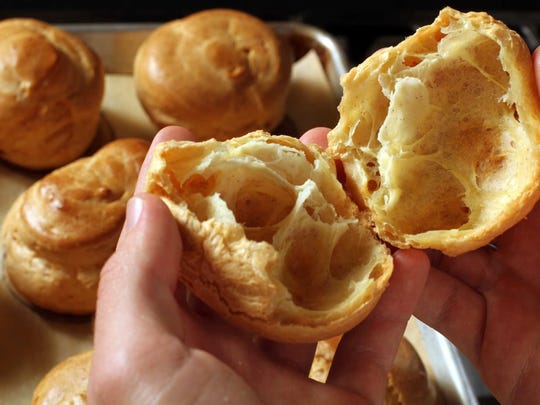A pair of Caucasian hands, smooth and well-kept, gently hold a golden-brown puff split in half, revealing its airy, hollow yellow interior. Below, on a silver rectangular tray lined with beige parchment paper, rest four to six freshly baked puffs, their crisp, tan exteriors glistening under the limited light. The dark, barely visible background accentuates the warmth and richness of the puffs, emphasizing their perfectly baked texture.